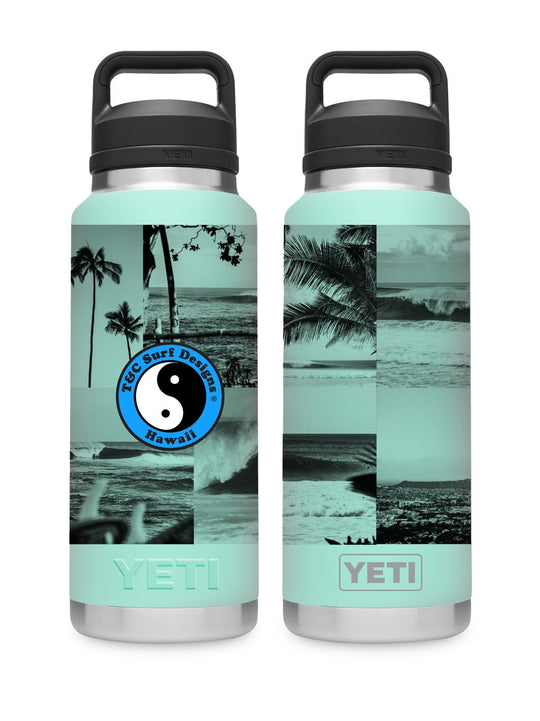The image showcases a pair of realistic photographs of stainless steel Yeti water bottles against a white background, displayed side by side, front and back. Both water bottles feature black lids with convenient handles. The left bottle prominently displays the TNC Surf Designs Hawaii logo in blue, centered with a yin yang symbol. The exterior of each bottle is artfully wrapped in a vibrant turquoise-colored image depicting a tropical beach scene, complete with black ink illustrations of palm trees, ocean waves, and faint impressions of Hawaiian civilization. The word "Yeti" is embossed on the bottles and also appears typed in either gray or aqua, enhancing the beach-themed design. The bottles' base is sleek, silver stainless steel, giving a polished contrast to the colorful, tropical decorations that evoke a sense of serene Hawaiian landscapes.